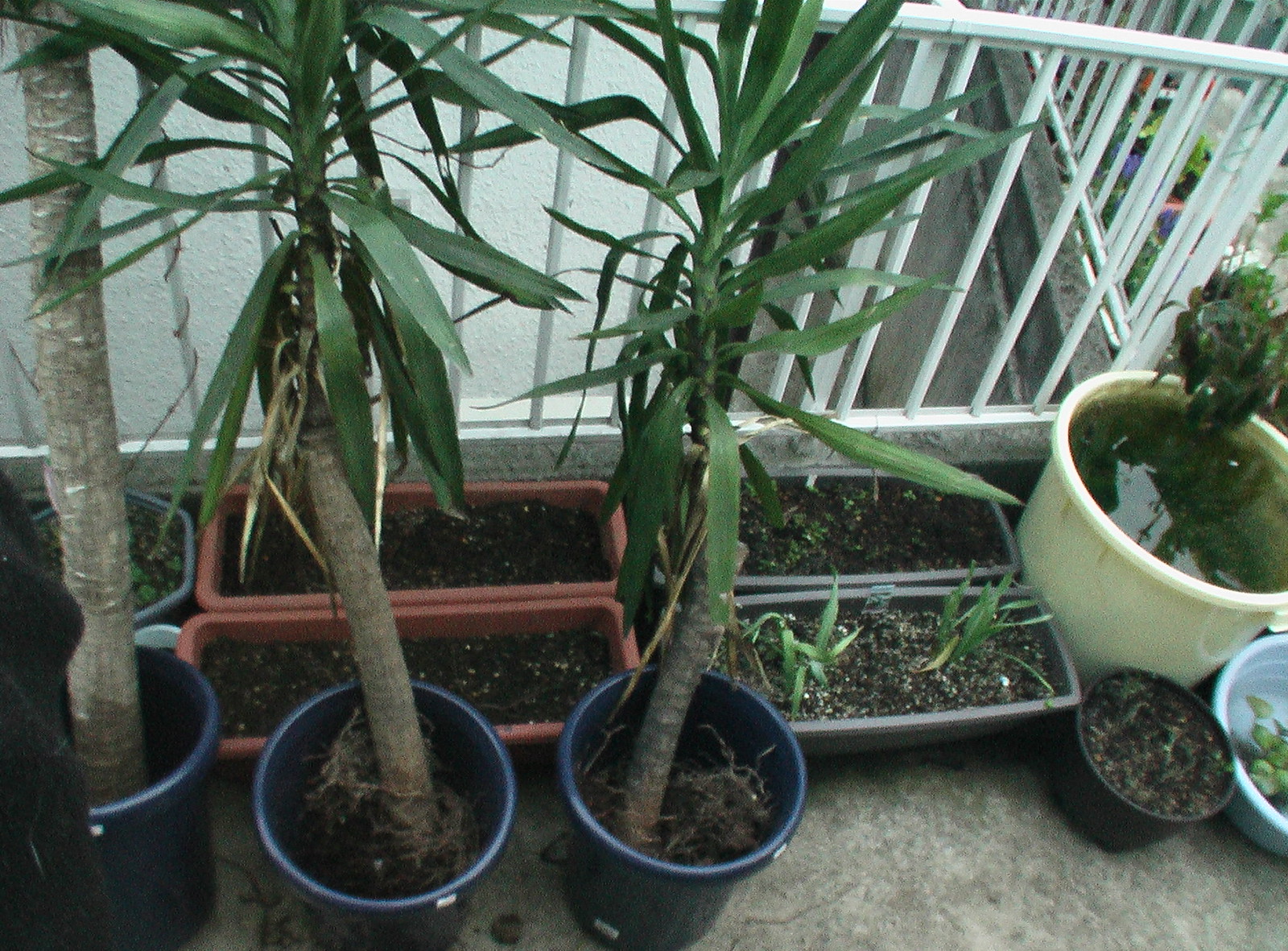The photograph depicts a garden area on a concrete patio or balcony, enclosed by a white metal rail fence. In the bottom left corner, three small trees with long, green leaves, resembling palm or banana trees, grow from dark blue plant pots. Behind these trees, there are four long rectangular planters: the two on the left are terracotta-colored, while the two on the right are gray. Only the gray planters contain visible plants, although they are too small to identify clearly. Toward the right side, the scene includes a variety of other pots: a small round black pot, a large round white pot that appears to be filled with greenish liquid, and a partially obscured small round blue pot with an unidentified plant. Additionally, there is a hexagonal gray pot on the left side, just visible behind the blue pots. Together, the array of pots and planters, along with their varied contents, suggest a diverse collection of plants and containers on this elevated outdoor space.